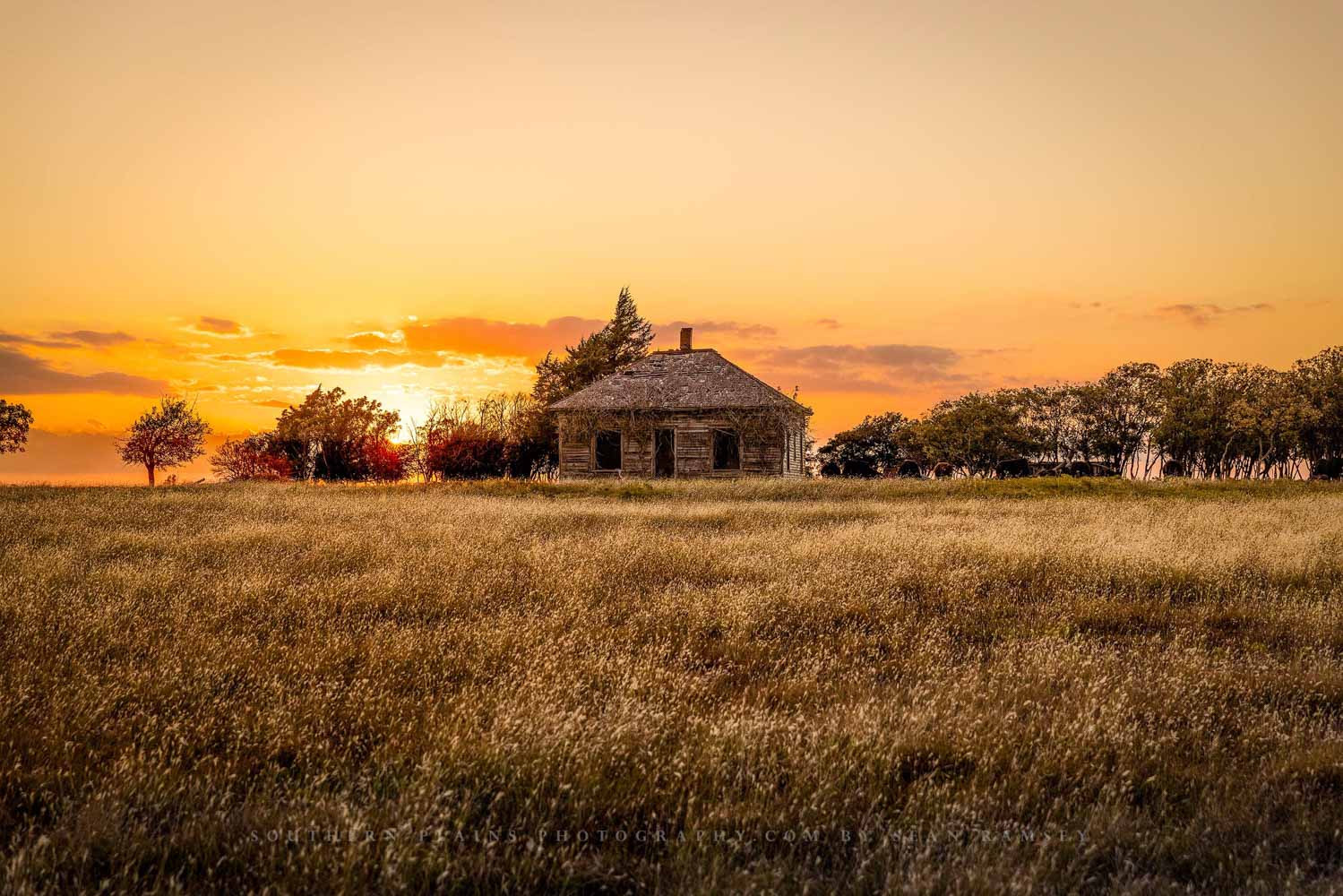This photograph, taken by Sean Ramsey of Southern Plains Photography, captures an old, abandoned log cabin situated in a remote and desolate area, blanketed by tall, amber grass that hints at the fall season. The cabin, primitive in style with a thatched roof and small chimney, stands solitary amidst a backdrop of trees. The sky is painted in mesmerizing shades of oranges, peaches, golds, and yellows, with the setting sun partially obscured by tree lines to the right and individual trees to the left. Dark, foreboding clouds accentuate the dramatic sunset. The cabin appears deserted, with dark windows and a door that beckon to its past life. The tranquil scene is completed with a distant hint of livestock, perhaps cows, contributing to the rustic charm of the Northern plains area.